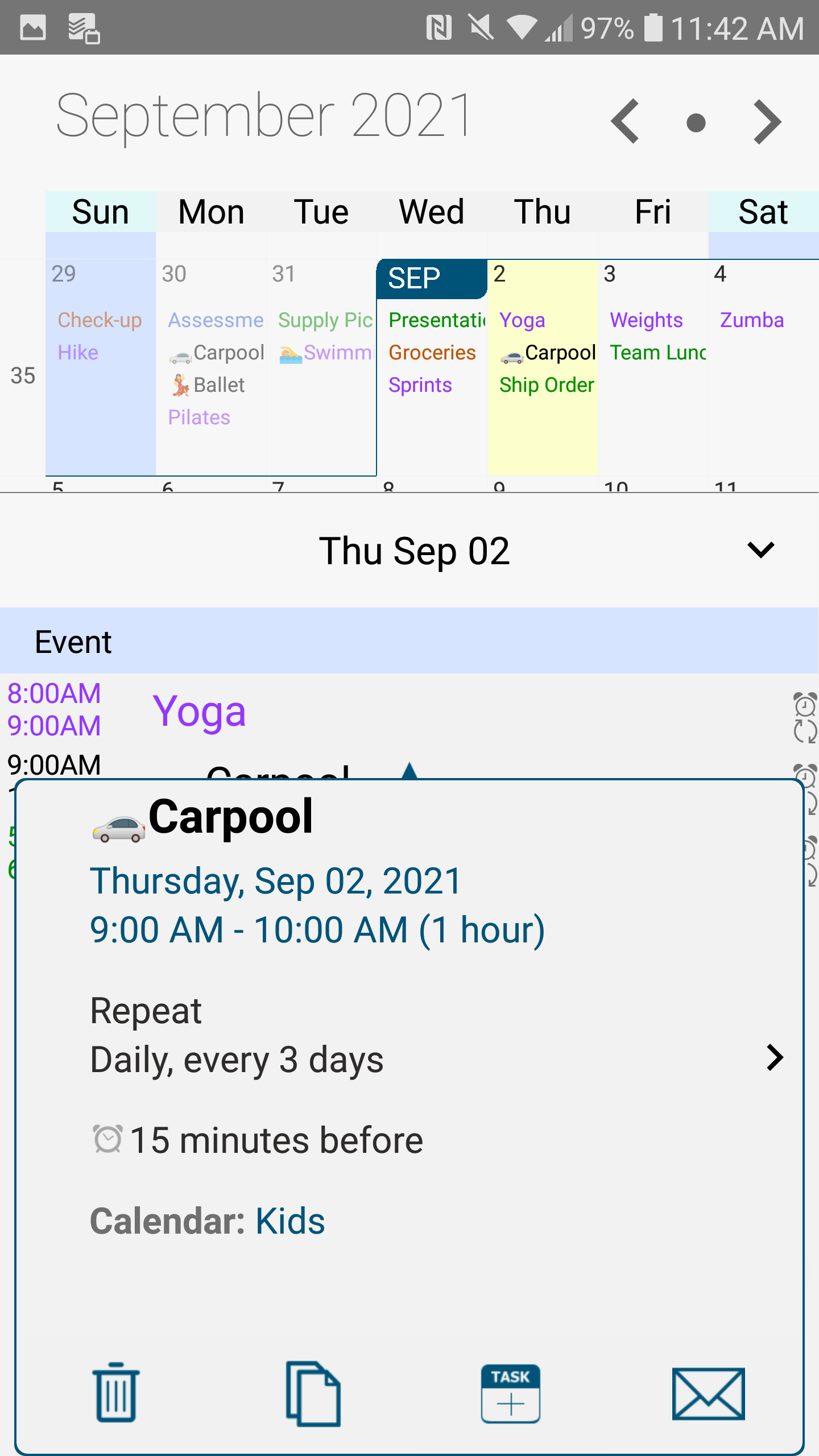The image appears to feature a digital calendar interface, resembling the screen of a smartphone. At the very top, the header mimics that of a typical cell phone status bar. Within the upper left-hand corner, two icons are visible: one resembles a map icon, and the other a download icon. To the right of these are additional icons indicating mute status, Wi-Fi connectivity, signal strength, battery percentage along with the battery icon, and the current time displayed as 11:42 a.m.

Below this header, the screen shows a calendar for September 2021, printed in a light gray text. The calendar is organized with the days of the week acting as headers above individual boxes for each day, starting from Sunday and progressing through to Saturday. Each daily box contains various events and scheduled activities. 

Highlighted specifically is Thursday, September 2nd. Within this date's detailed view, events are broken down into hourly increments. An entry from 8:00 to 9:00 a.m. is labeled "yoga," followed by another entry labeled "carpool" with a card icon to the left. This "carpool" event reads: 
"Thursday, September 2nd, 2021, 9 a.m. to 10 a.m., one hour,
  repeat daily, three days, 
  15 minutes before, 
  calendar: kids."

At the bottom of the screen, there are four icons aligned to the left. From left to right, these include a trash can icon, an overlapping papers icon, a task button, and finally, an envelope icon typically representative of email, located in the bottom right-hand corner.